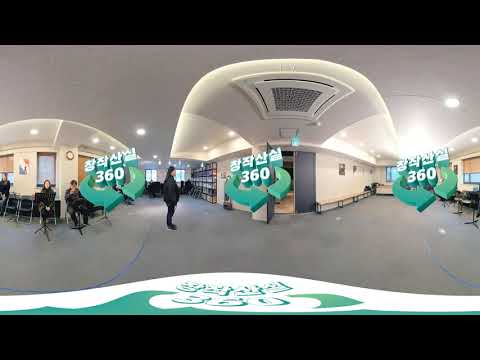This image captures a 360-degree interior view of a predominantly white-walled building, possibly an office or a store. Three floating symbols featuring four Asian characters (likely Korean) and the number "360" are prominently displayed, indicating the 360-degree nature of the view. Below the leftmost symbol, three people are seated on black chairs, facing the camera. To the left of the central symbol, a person dressed in all black stands, looking to the right. On the right side, there is notable empty space with no furniture or people. The ceiling is equipped with a vent featuring numerous small holes, projecting slightly from the ceiling's plane, and the floor appears to be covered in a white carpet. The ambiance includes spotlights on the ceiling, adding to the well-lit, spacious feel of the room, while the walls possess a light yellow hue, enhancing the overall brightness of the space. The arrangement of the symbols and arrows further implies an interactive VR experience, emphasizing the 360-degree perspective.